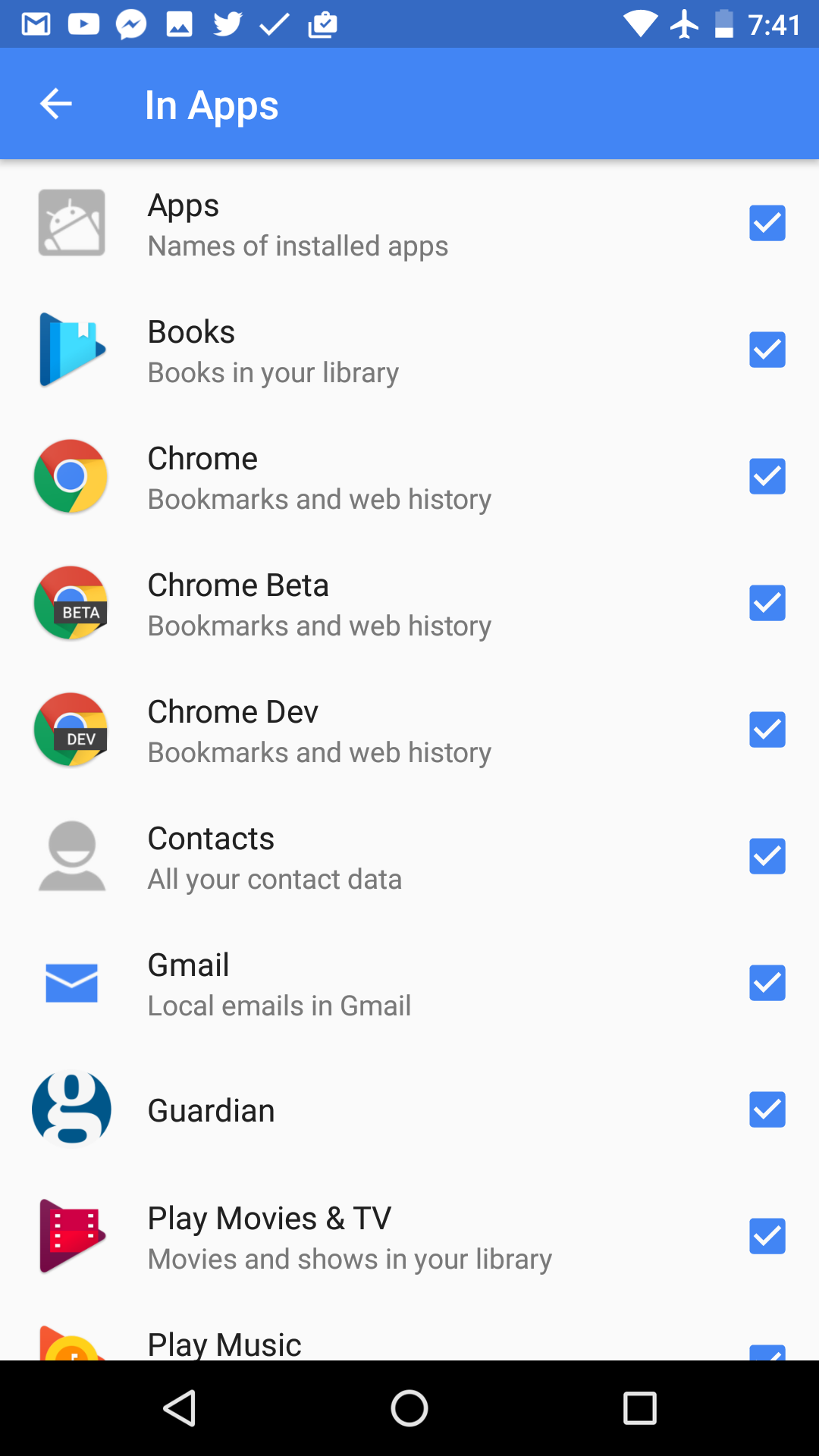This image is a screenshot taken from an Android mobile device, identifiable by the navigation buttons at the bottom: a backward-facing arrow for back, a circular home button, and a square to open recent apps. The main screen is displayed in the settings section of an app, featuring a blue header at the top labeled "In-Apps," with a left-facing arrow to return to the previous page.

Below the header, the screen lists several apps in a vertical sequence, each accompanied by a checkbox on the right side, all of which are currently checked with white checkmarks against blue backgrounds. The listed apps and corresponding descriptions are as follows:

1. **Apps** - Names of installed apps.
2. **Books** - Books icon: Books in your library.
3. **Chrome** - Google Chrome icon: Bookmarks and web history.
4. **Chrome Beta**
5. **Chrome Dev**
6. **Contacts**
7. **Gmail**
8. **Guardian News** - Guardian News website.
9. **Play Movies & TV** - Google Play Movies and TV.
10. **Play Music** - Google Play Music.

This detailed screenshot provides a comprehensive view of the selected apps within the "In-Apps" settings section on an Android device.